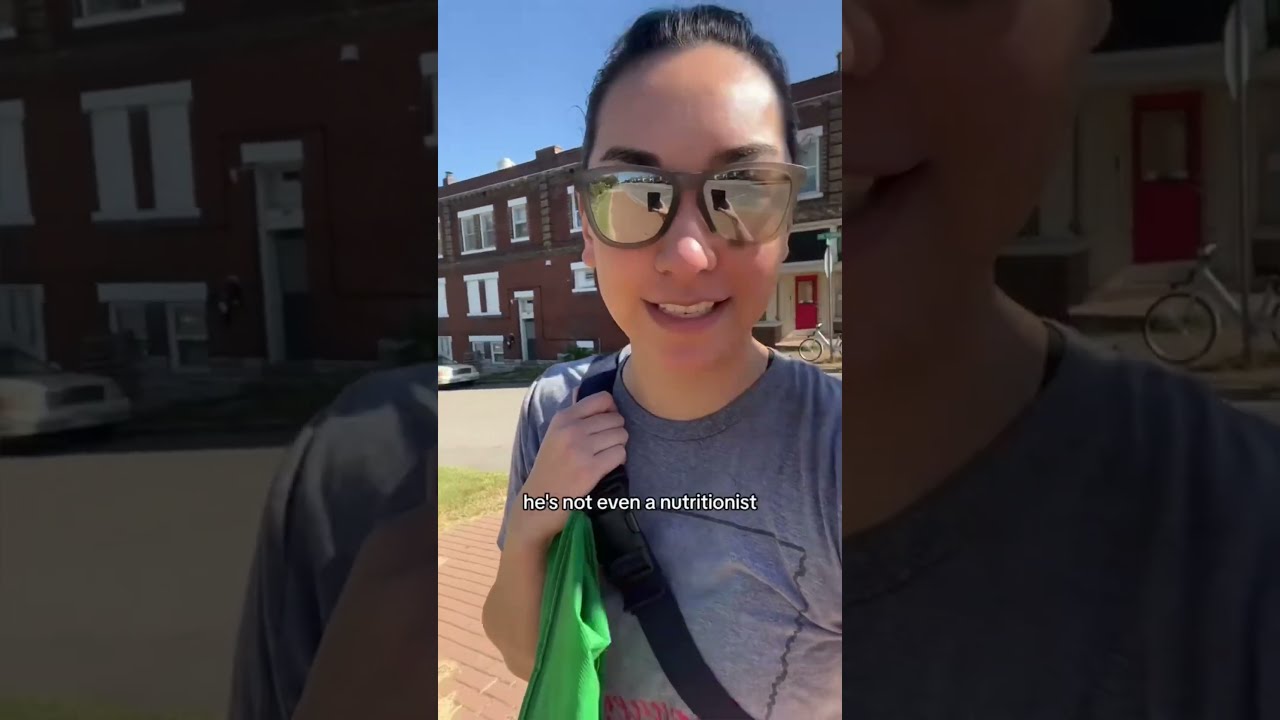The image is a detailed and vibrant screenshot of a young woman, seemingly around 20 years old, possibly of Asian descent, taking a selfie video, likely for an Instagram reel or similar app. The image is split into three panels. The central panel is in full color, showing the woman, who has her hair swept back and is partially smiling, standing outdoors against a backdrop of a two-story apartment building with distinctive red and brown accents. The left and right panels are zoomed-in, close-up shots of her face. She wears large reflective sunglasses that mirror the phone she is holding up to her face. She dons a dark gray shirt, accessorized with a black crossbody strap and carries a green bag over her shoulder. In the middle of the image, white text overlays her body, reading "he's not even a nutritionist," suggesting she is reacting to some surprising information. The background also includes a parked white car, a bicycle, and a backwards stop sign.